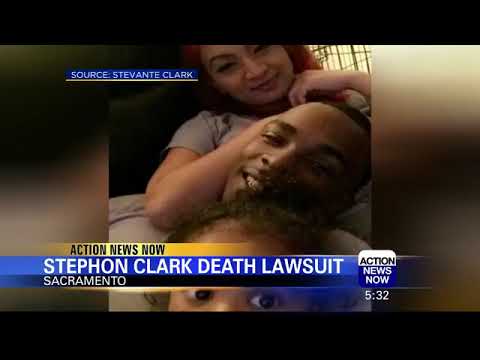The image appears to be a screen grab from a news report, focusing on a family selfie that is being used to illustrate a story about the Stephen Clark Death Lawsuit in Sacramento. The banner at the bottom reads "Action News Now, Stephen Clark Death Lawsuit, Sacramento" and indicates the time as 5:32. The central figure in the image is a young African-American man, presumably Stephen Clark, who is lying down and smiling, with short hair. Behind him, a woman with red hair, likely his wife or girlfriend, is holding his head and also smiling. In front of Stephen, a child, possibly their son or daughter, is looking off to the side, with only the upper part of their face visible. The overall impression is of a loving and happy family, despite the tragic context suggested by the news banner.